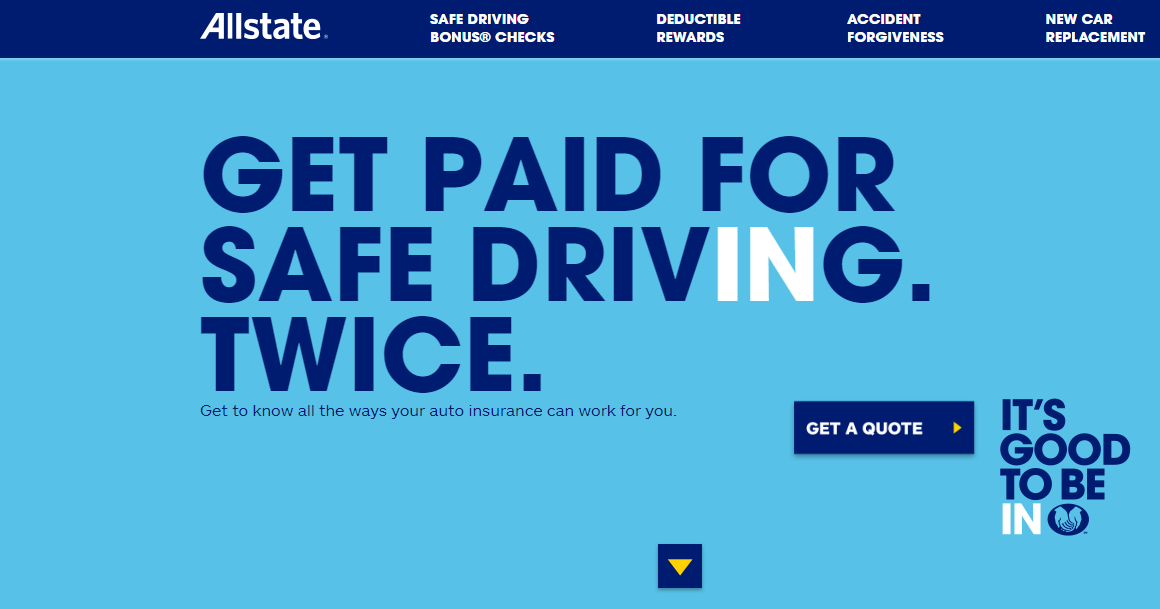A detailed webpage designed for an auto insurance company is displayed, featuring a prominent navy navigation bar at the top with white clickable options: "All States," "Safe Driving Bonus Checks," "Deductible Rewards," "Accident Forgiveness," and "New Car Replacement." Below the navigation bar, a large light blue background dominates the page, with various font colors used for emphasis and readability.

Central to the page, in bold navy text, is the message "Get Paid for Safe Driving Twice," drawing attention with the word "IN" in white to highlight part of the text. Beneath this, another navy text reads, "Get to know all the ways your auto insurance can work for you," providing further information. 

A prominent navy box contains white font stating "Get a Quote," accompanied by a striking gold button for user interaction. Below this, a navy and white slogan, "It's Good to be IN," is featured, alongside a navy circle icon with light blue hands, symbolizing care and support.

At the very bottom, a small blue box with a gold down arrow is present. The webpage is clean and easy to read with no pixelation or blurring, boasting excellent readability due to the large font size used throughout. The design is straightforward with no other images or additional elements of note.